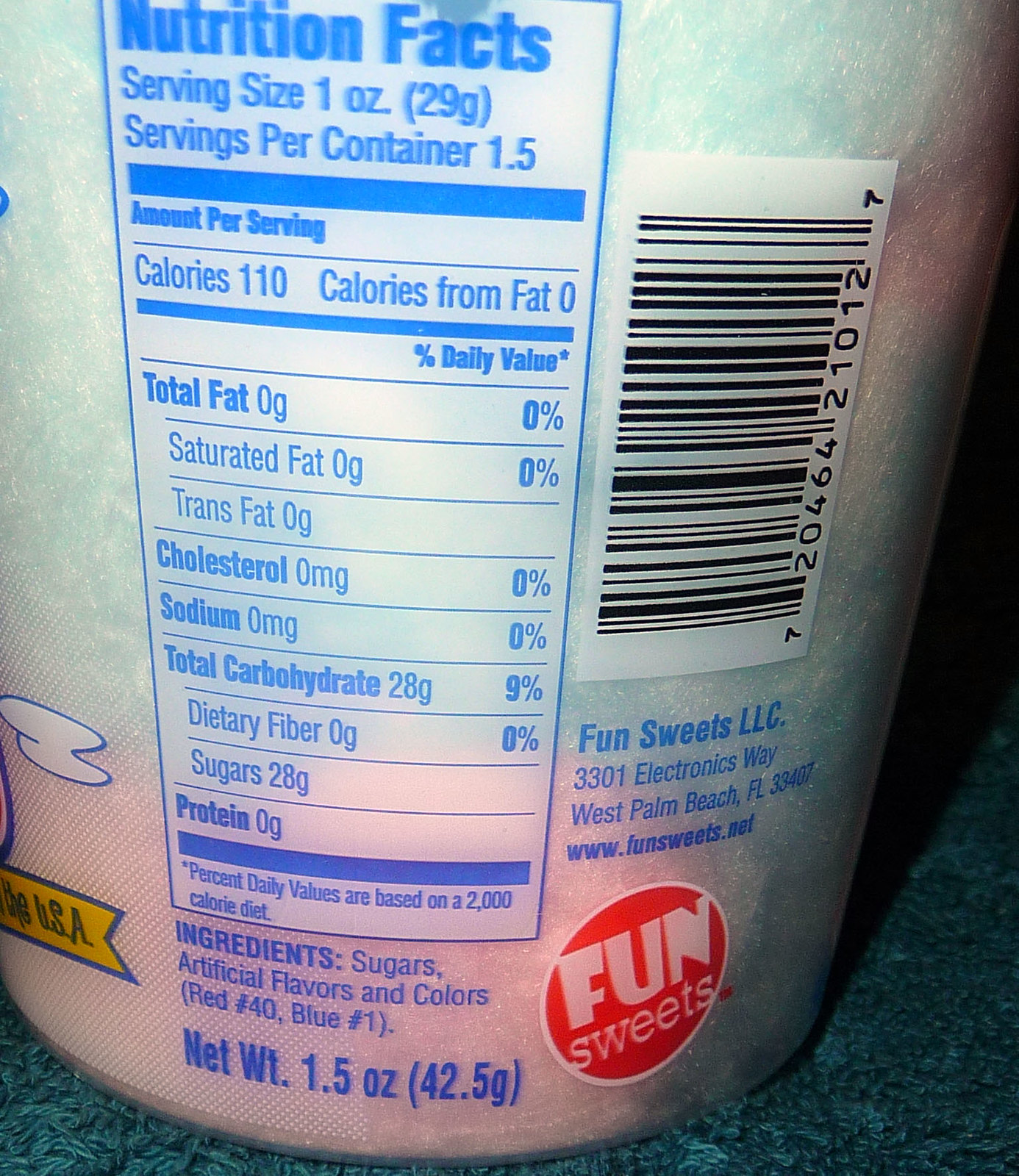This close-up, portrait-oriented photograph captures the backside of a rectangular canister of cotton candy. The vibrant interior of the canister reveals fluffy swirls of bright blue and light pink cotton candy. The focal point of the image is the detailed nutrition label, which is printed in a dark blue font. The label includes nutritional information and ingredients, prominently displayed. Alongside it, on the right side of the canister, a barcode can be seen. At the bottom right corner, the Fun Sweets LLC logo is elegantly enclosed in a red circle, with the brand name "Fun Sweets" boldly written in white font. The overall composition and colors of the photo create an enticing and informative visual experience.